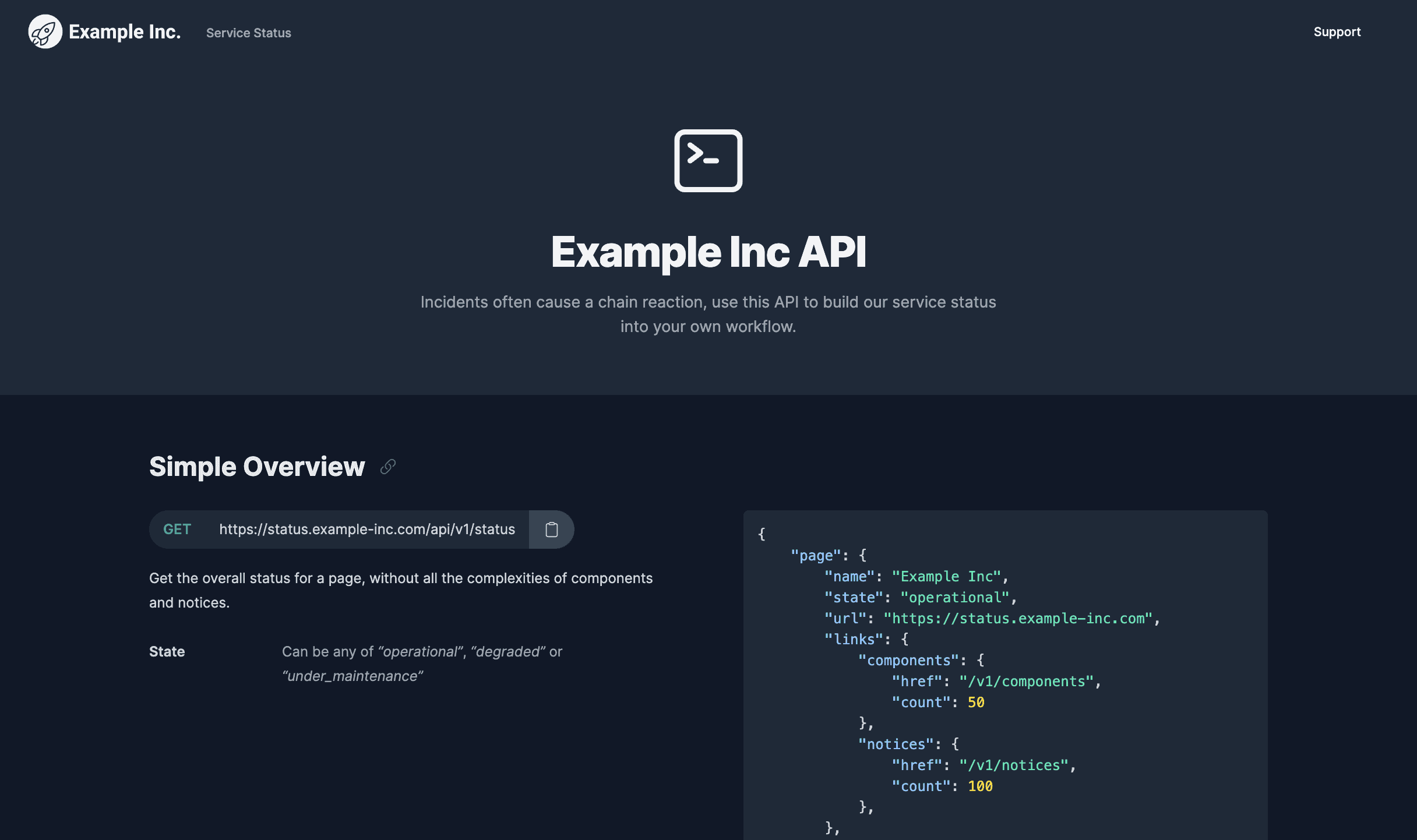### Detailed Descriptive Caption

This image depicts a complex application interface on a predominantly black background. At the top of the page, white text introduces the scene, accompanied by a logo featuring a whitish-gray circle with a simple, crudely drawn black rocket ship in its center. Beside the logo, the text reads "Example Inc.," followed by a smaller note in gray indicating "Service Status." On the right-hand side, there is a button labeled "Support."

The central section of the page features a lighter black background with a square box containing the word "Open" followed by a dash, suggestive of an operational status indicator. Below this, it mentions "Example Inc. API," with an explanation in gray text that states, "Incidents often cause a chain reaction. Use this API to build our service status into your workflow."

Further down, the page transitions back to a very dark black background. On the left-hand side, "Simple Overview" is displayed in white text, accompanied by a gray chain link icon. Below that, there is a gray button labeled "Get," near the website status URL "status.example-inc.com." A descriptive text follows in white, advising the user that this API can provide the overall status of a page without delving into the complexities of components and notices. The possible states are listed in gray as "Operational," "Degraded," or "Under_Maintenance."

To the right, set against a gray background, some sample coding is presented. Each line of code begins in blue with parentheses and ends in white text, barring two lines. One line containing "count" concludes in green with the number "50," while another ends with "count" marked in green with the number "100." The coding area emphasizes the API's capabilities in returning status counts.

This detailed interface captures the essence of a functioning Service Status API dashboard, presenting both visual and textual elements thoughtfully aligned for clarity and user engagement.